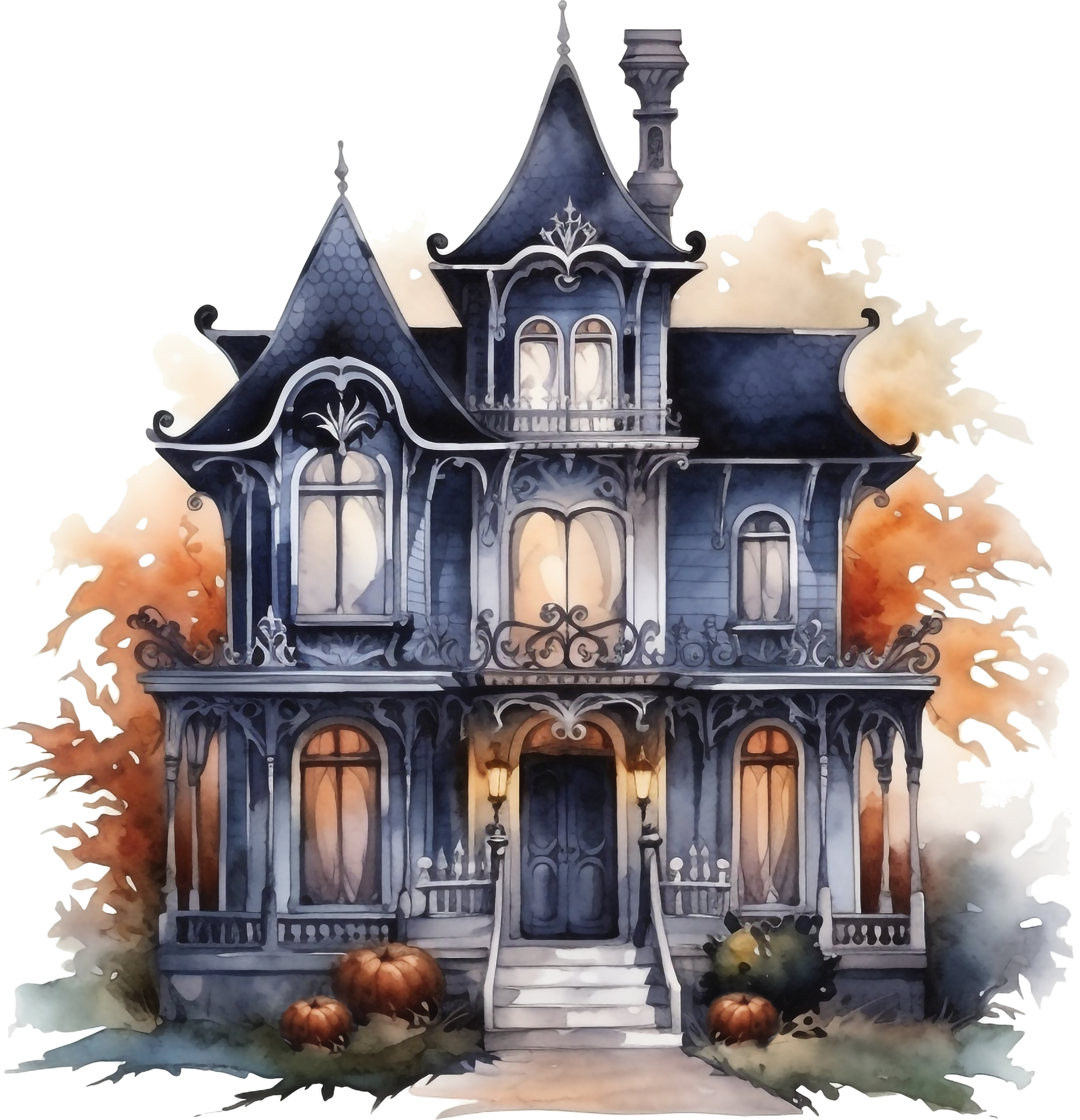The image depicts a detailed watercolor painting of an old Victorian-style house, predominantly in bluish gray with white woodwork. The house features a dark, bluish-gray roof and a chimney. It stands two and a half stories tall and has a distinct haunted or Halloween-themed ambiance. The front of the house has four steps leading up to a porch with vintage-style railings and arches.

The front door is double and black, flanked by two orange vintage lights. Surrounding the door are two windows on the ground floor, while the second story has three windows—one in the center and two on either side. The half-story attic, resembling a small tower at the center, hosts a pair of double windows.

The front yard showcases three orange pumpkins, with two positioned on one side of the steps and one on the other, and a small shrub nearby. The background hints at a festive atmosphere with orange frilly decorations emerging from behind the house, enhancing the Halloween theme. Overall, the house exudes an older, slightly eerie charm enhanced by its vivid decoration and careful details.